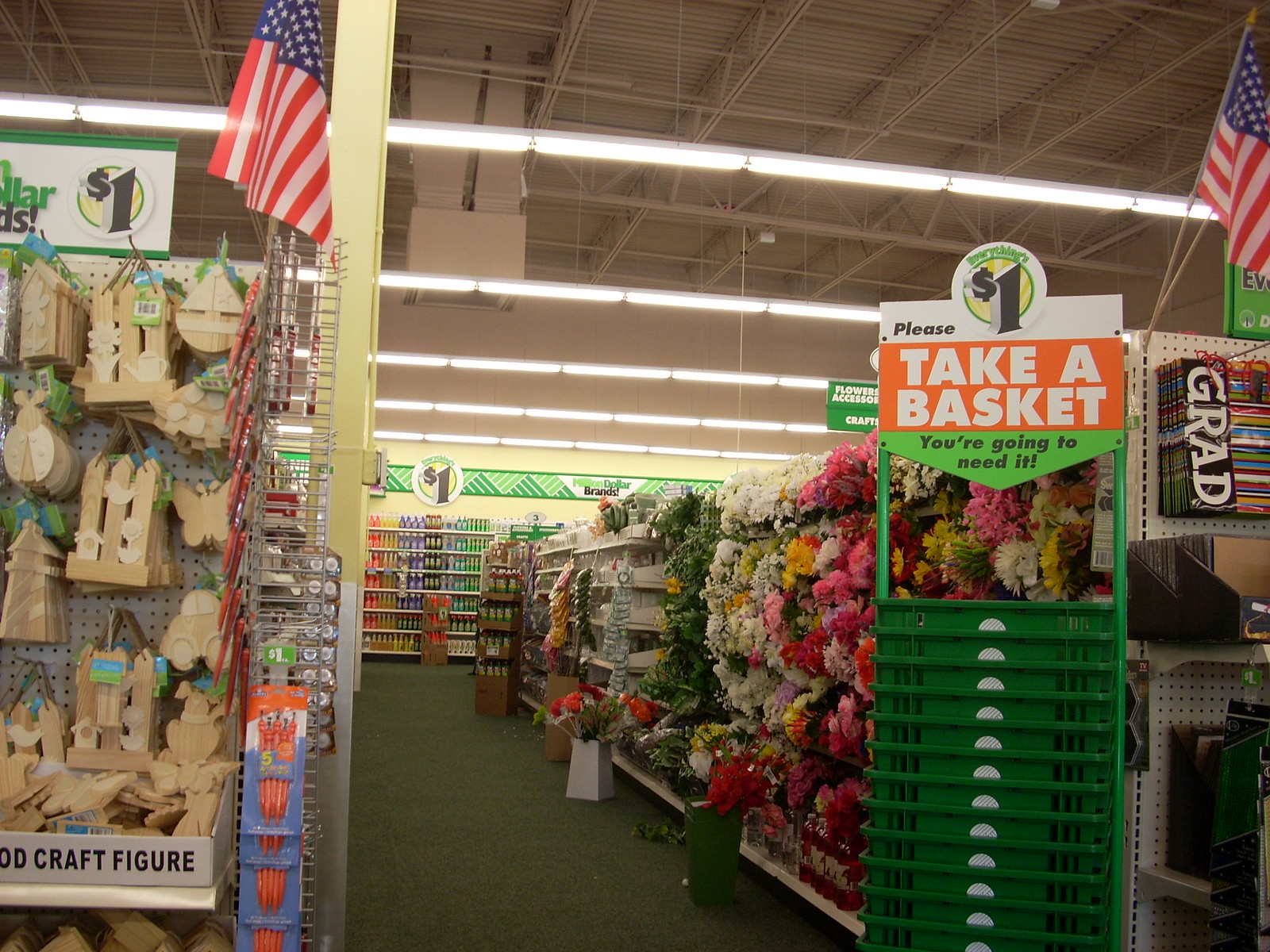The image depicts the interior of a dollar store, resembling a Dollar Tree. The ceiling has a warehouse style with white metal panels, steel beams, and fluorescent lights running across it. In the foreground, there's a stack of green shopping baskets with a sign that says, "Take a basket, you're going to need it." The aisle visible starts with various unpainted wooden ornaments along a white pegboard on the left, labeled "craft figure." On the right side of the image, shelves display a range of colorful items, fake flowers, and bottles. At the far end of this aisle, the wall at the back of the store features a prominent dollar sign ($1) high up. Additionally, towards the end of the aisle, there are shelves stocked with drinks and jars of different colors. On the right, there are small American flags for sale and some graduation-themed gift bags, one of which has "grad" written on it. The carpet along the aisle is green, complementing the overall color scheme of the baskets.